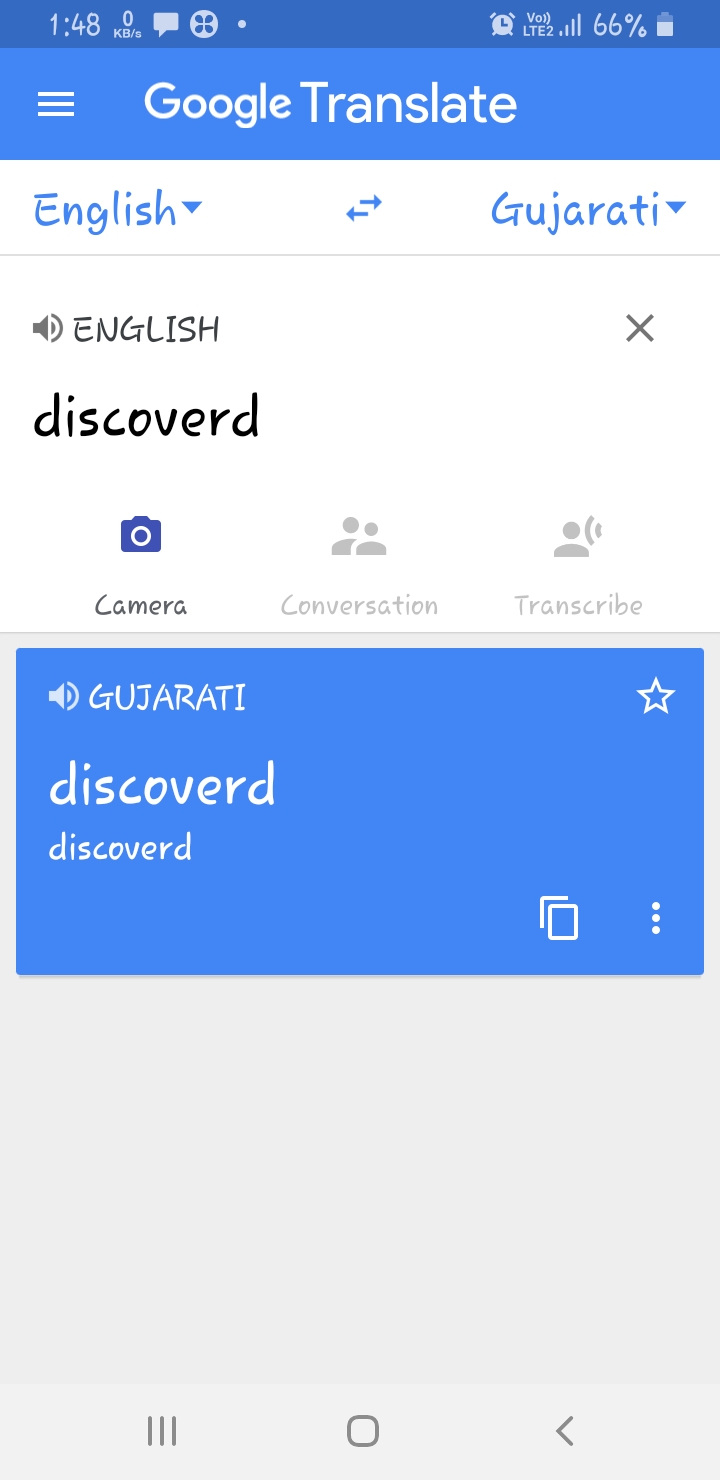A detailed smartphone screenshot captures a moment at precisely 1:48. At the top of the screen, several icons are visible: a white logo symbolizing an ongoing conversation, an alarm clock icon, a signal strength indicator showing four bars, and a battery icon indicating a 66% charge. 

Dominating the top section, a blue banner displays "Google Translate" in bold white letters. The translation settings are set from English to Gujarati, with English currently selected. A speaker icon next to "English" is marked with an X, indicating it is muted.

Below the language selection, the word "Discovered" appears prominently. Towards the middle of the interface, three buttons are lined up: a camera icon (highlighted in blue), a conversation icon, and a transcribe icon. 

Further down, a speaker icon indicates the pronunciation feature for Gujarati, accompanied by a star icon meant for favoriting the translation. The word "Discovered" reappears, maintaining the same format and font. The bottom of the screen features several navigation tabs, completing the layout of this detailed screenshot.